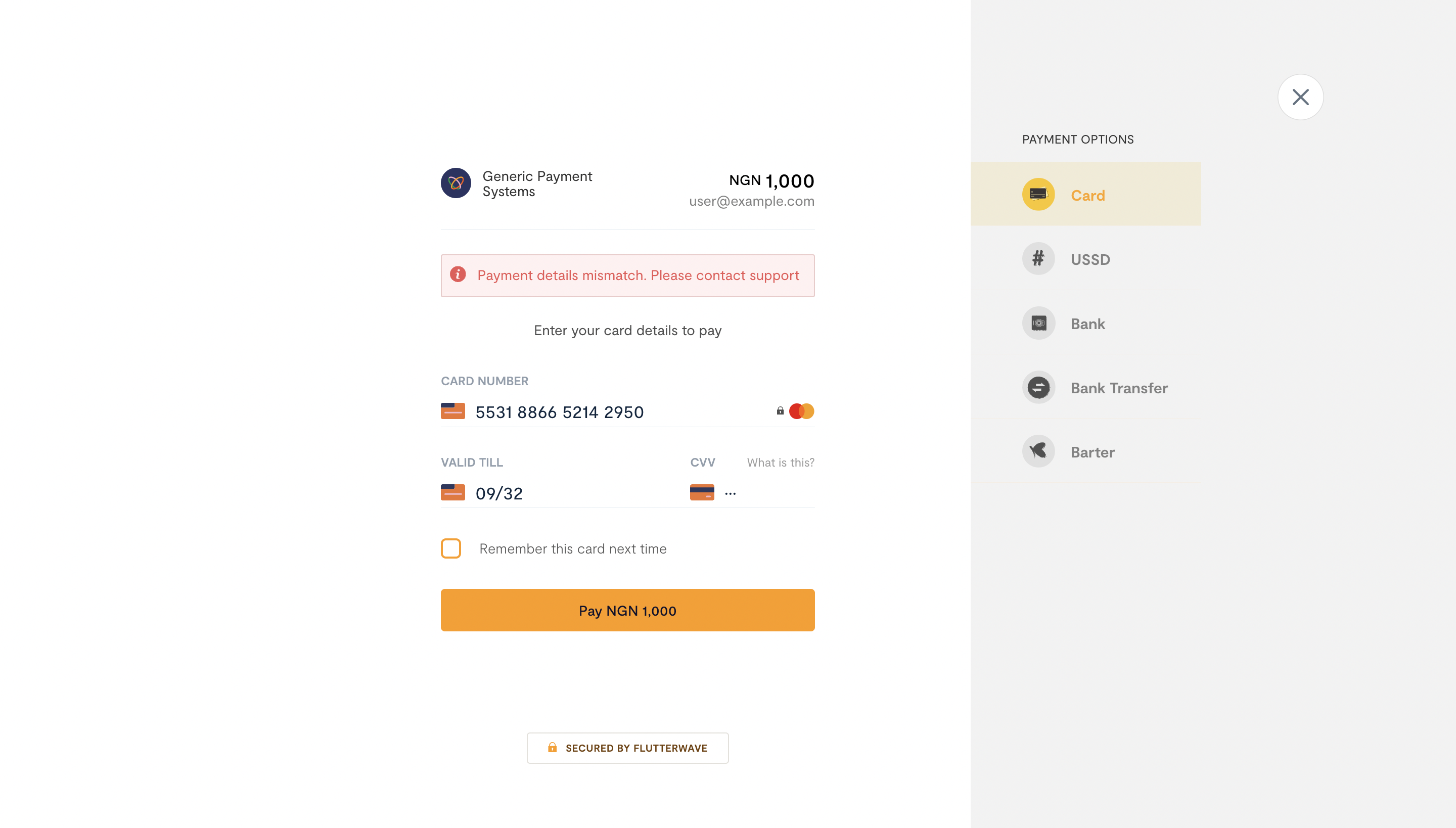This desktop screenshot depicts a user interface for a payment processing system. The left side of the screenshot features a predominantly white background, displaying the heading "Generic Payment Systems" accompanied by a company logo to its left. Adjacent to the heading, the amount "NGN 1000" is indicated. Below, the text "user@example.com" is shown, followed by a light pink rectangular box containing the error message in red text: "Payment Details Mismatch. Please contact support."

Further down, the interface prompts the user to enter their card details with the instruction "Enter Your Card Details to Pay." A card number field is filled with "5531-8866-5214-2950," displaying a US flag to its left and the MasterCard logo to its right, along with a small padlock icon. Directly underneath, the card's expiration date "Valid till 09/32" is displayed, along with a blank CVV field followed by a "What is this?" link providing additional information about the CVV.

An orange square checkbox offers the option to "Remember this card next time." At the bottom, an orange rectangular button invites the user to "Pay NGN 1000." The interface is secured as indicated by a white rectangular box at the very bottom that reads "Secured by Flutterwave."

On the right half of the screenshot, payment options are listed, with "Card" being selected. Other payment options include "USSD," "Bank," "Bank Transfer," and "Barter." At the extreme top-right corner, a white circle encloses a black X mark, likely functioning as a closeout button for the interface.